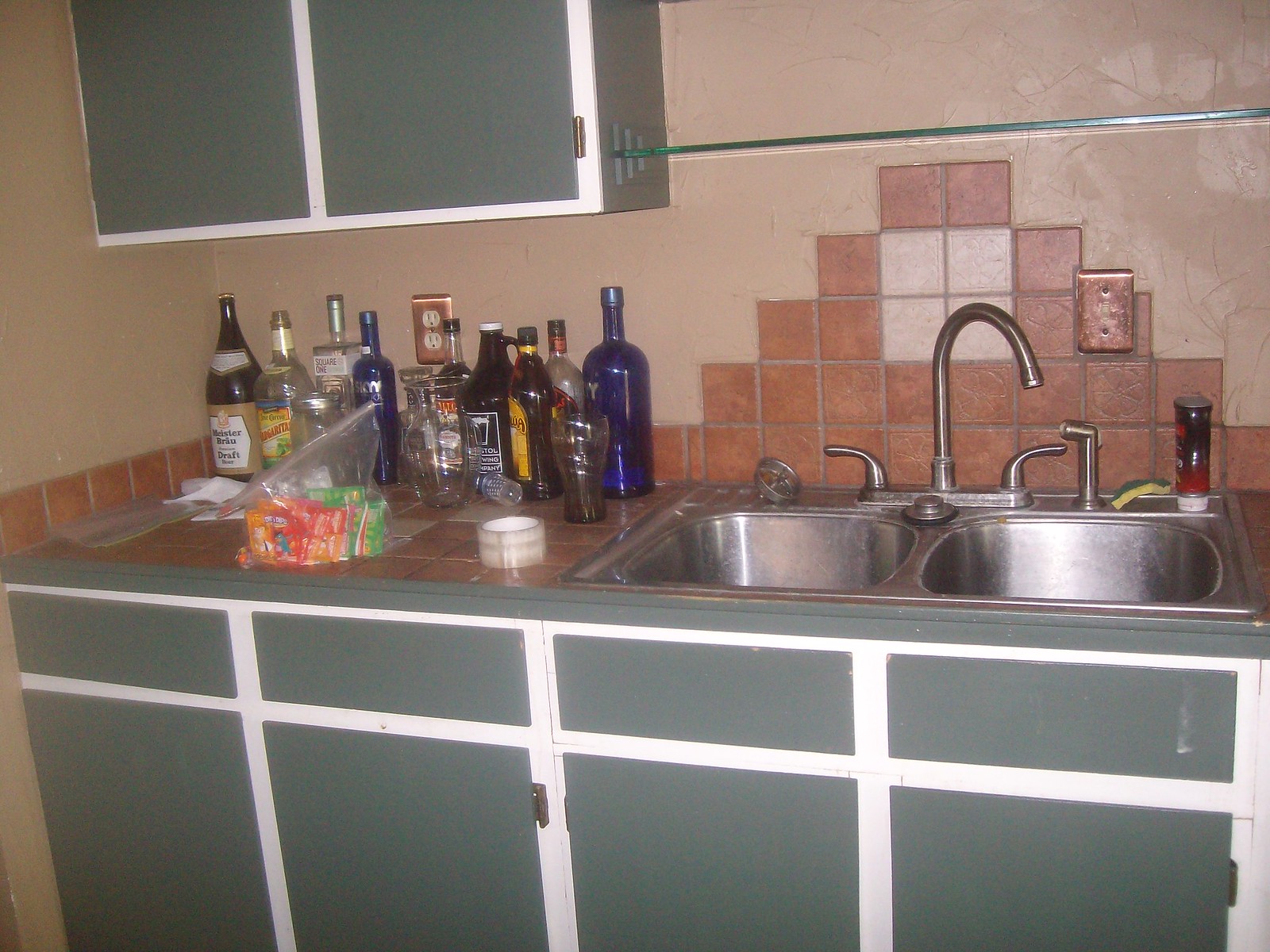This photo captures a well-used kitchen sink area with a hint of rustic charm. The cabinetry is predominantly painted a soft green, accented by white outlines that delineate the edges, giving the kitchen a fresh, inviting look. Each cabinet door features the same muted green, reinforcing the cohesive color scheme.

The countertop is adorned with square tiles in earthy tones ranging from orange to brown, creating a warm, textured surface. The wall above the counter is painted a much lighter shade of brown, almost bordering on tan or peach, adding a gentle contrast to the richer hues below.

Positioned to the right is a silver sink with twin basins and traditional twist handles, complemented by a handy sprayer attachment. To the left of the sink, a collection of glass bottles, likely containing alcohol, is clustered together, suggesting a touch of festivity or culinary experimentation. Behind these bottles, an electrical outlet is subtly visible, hinting at the practicality integrated into the kitchen’s design. Additionally, a plastic bag containing packaged items adds an element of everyday life to the scene, emphasizing the kitchen’s role as a functional and lively space.